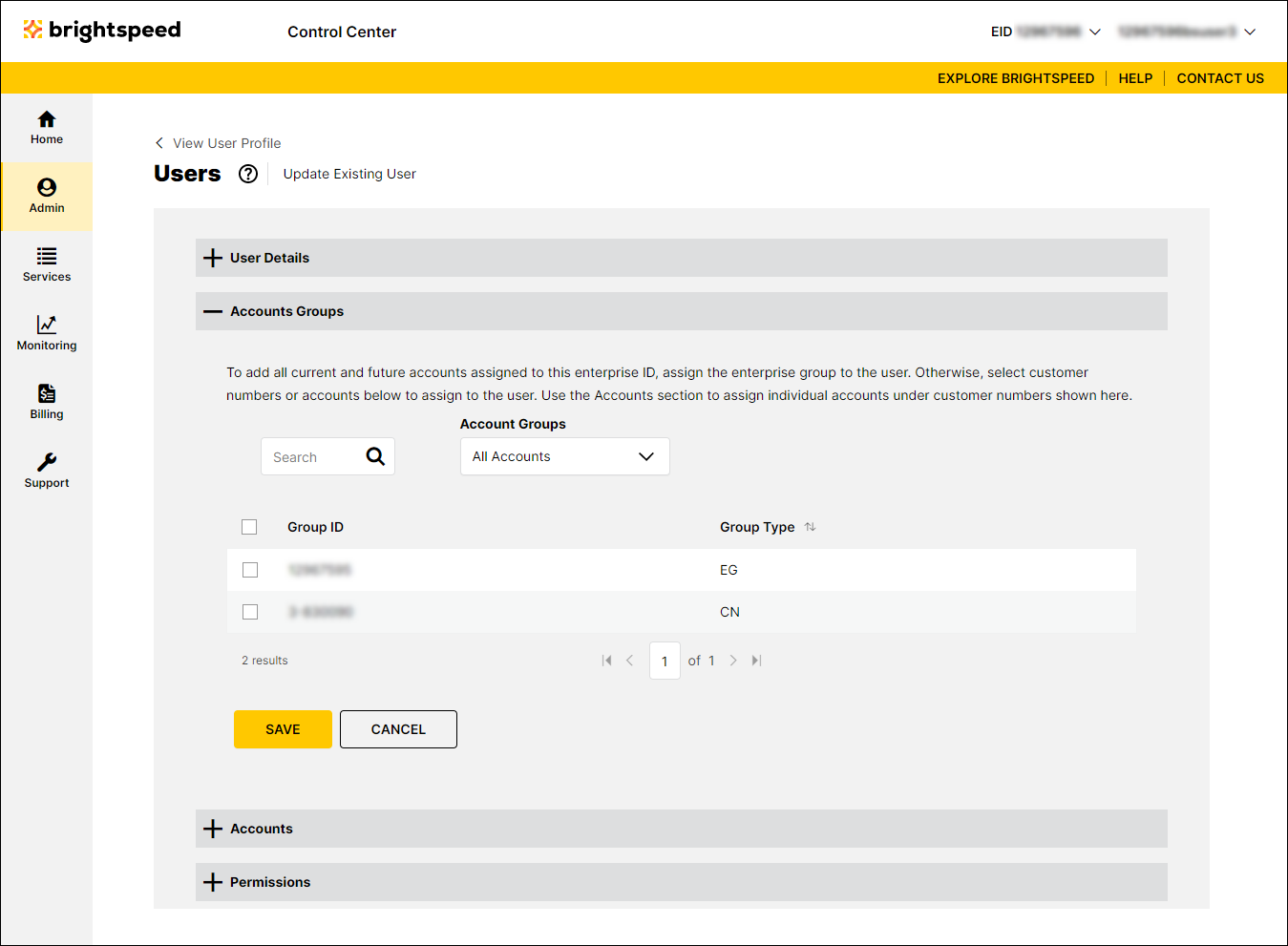Screenshot of the BrightSpeed Control Center interface. The BrightSpeed logo is prominently displayed in yellow and orange on the left side, with the word "BrightSpeed" next to it in lowercase black text. To its right, "Control Center" is written in a grayish-black color, not bolded. On the same horizontal line to the far right, an EID is blacked out, followed by a dropdown menu that is grayed out and unreadable.

Directly below, there's a gold navigation bar featuring options: "Explore BrightSpeed," "Help," and "Contact Us" on the right side. The left sidebar displays navigation links including "Home," "About," a menu icon (resembling a stack of pancakes) for additional options, "Monitoring," "Billing," and "Support." The interface is currently focused on the second navigation link under "User Profile," specifically on the "Admin" section displaying "View User Profile" in bold text.

Below, there's a form titled "Update Existing User" for modifying user details, followed by sections for "Accounts" management, "Account Groups," and related options. Users can perform tasks such as saving, canceling, adding accounts, or modifying permissions through the interface.